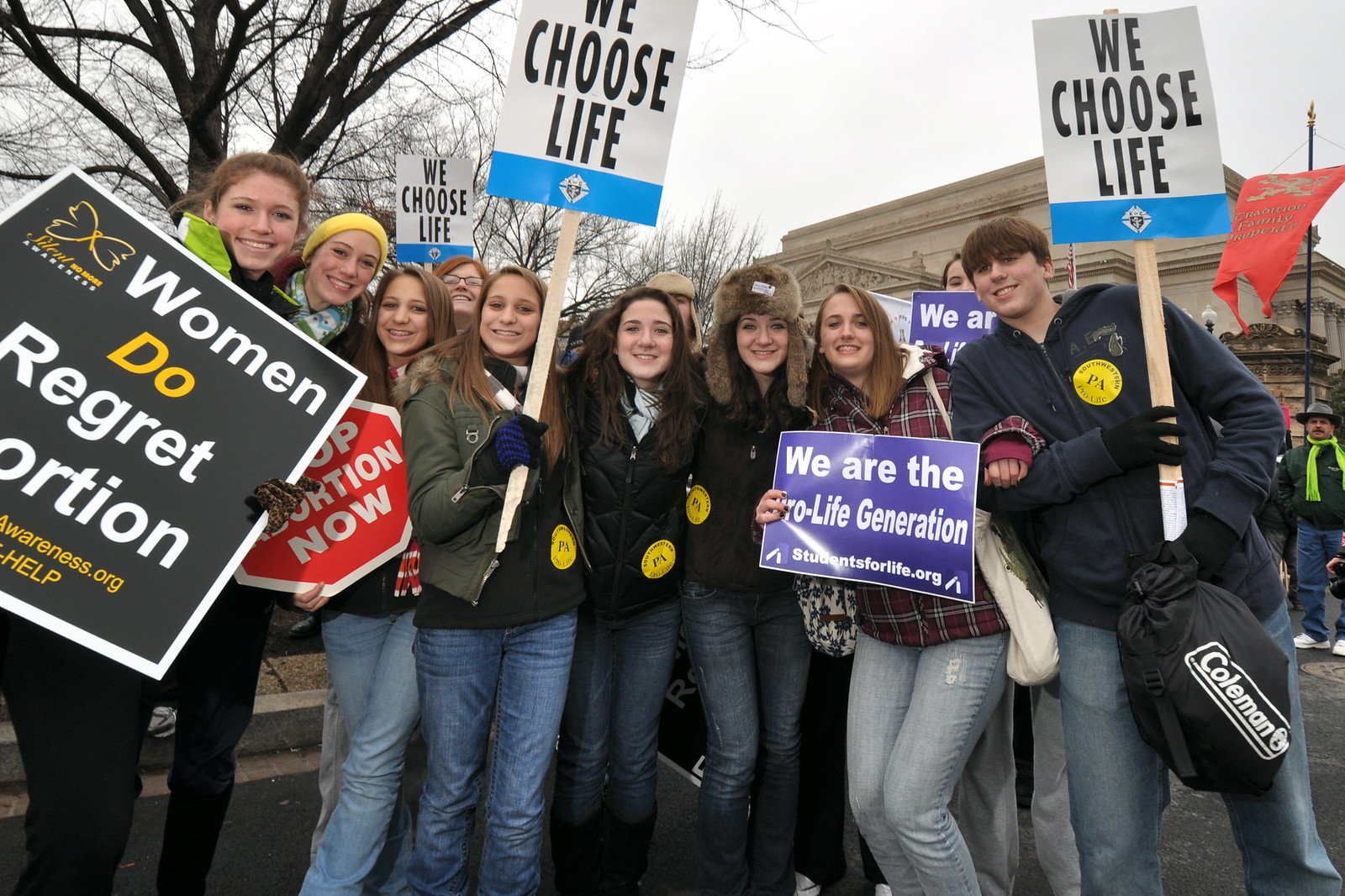The image is a color photograph in landscape orientation, capturing a vibrant scene of a group of young people participating in a pro-life protest. They are standing side-by-side, smiling and posing for the photograph, showing a sense of unity and enthusiasm. On the far left, a girl in a yellow reflective jacket and black pants holds a black sign with white lettering that reads, "Women Do Regret Abortion." Next to her, a woman wearing a black coat, a yellow beanie, and black pants holds a sign designed like a stop sign that says, "Stop Abortion Now." Moving towards the right, another girl in blue jeans and a black jacket stands next to a girl in blue jeans, a green jacket, a black shirt, and a black and white plaid scarf, holding a wooden pole with a white and blue sign that reads, "We Choose Life." Further to the right, a girl also in blue jeans and a black jacket completes the group of young women forming the core of the image. 

In the middle, some individuals are not holding signs but are still engaged in the group moment. As you look toward the right side, there is a girl holding another sign that reads, "We Are the Pro-Life Generation," and a man next to her holding a similar "We Choose Life" sign, with a black Coleman bag in his left hand. The background reveals several buildings and leafless trees, indicating a late autumn or winter setting. An orange pennant banner is seen in the upper right corner. The style of the photograph is representational realism, vividly capturing the moment and emotions of the participants.